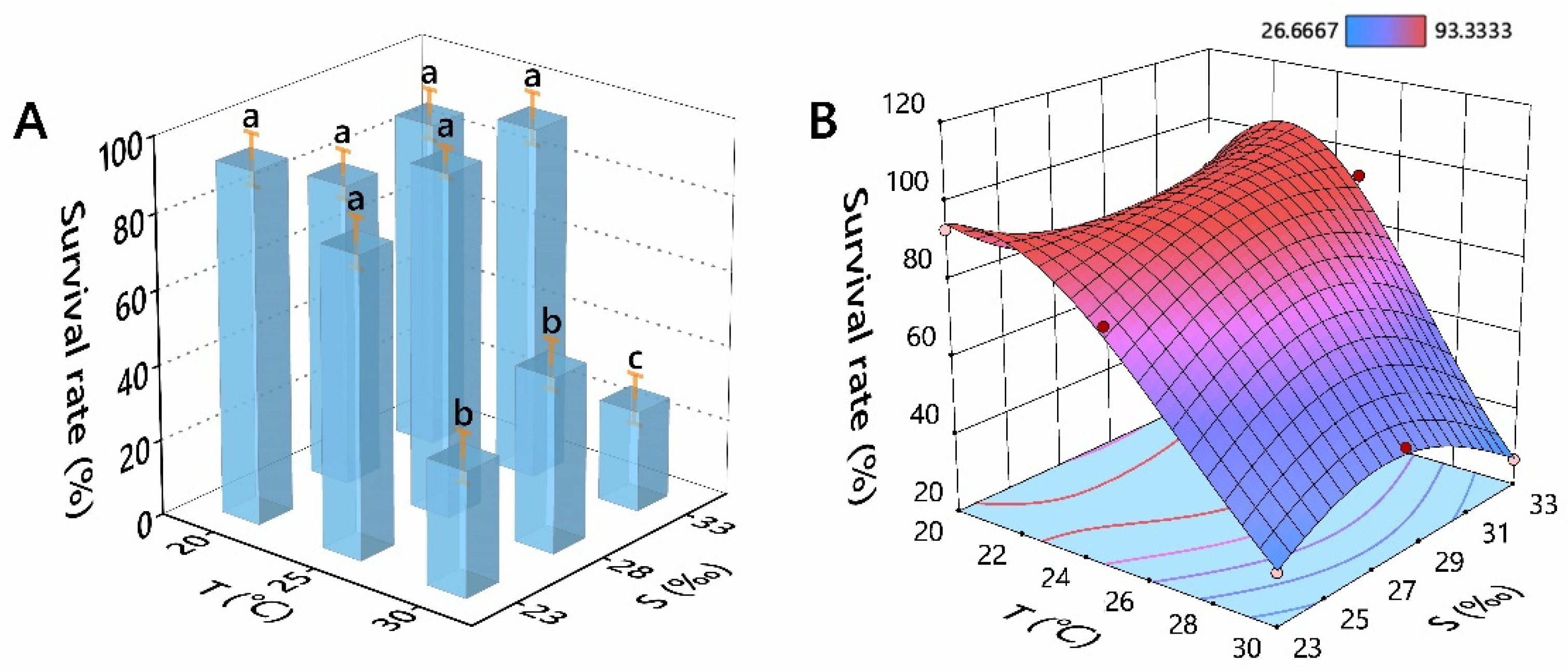This image showcases two distinct 3D graphs, labeled as Graph A on the left and Graph B on the right.

Graph A features vertical 3D rectangles set on a grid, representing survival rates. The axes are labeled with Celsius on the vertical axis and an unspecified "S" on the horizontal axis. Each rectangle is topped with the Amazon logo, indicating perhaps a comparative analysis of different data sets. The height of the rectangles varies: the tallest rectangles are labeled "E," the medium-height rectangles are labeled "B," and the shortest rectangle is labeled "C."

Graph B displays a textured surface graph with a gradient coloration ranging from red to purple to blue. This graph also includes a blue base grid with red lines running across it for reference. The axes in Graph B are labeled as survival rate on the X-axis and have the same vertical and horizontal labels of Celsius and an unspecified "S" as in Graph A. The graph appears to depict more complex, continuous data, and interpreting it might require a deeper understanding of the provided metrics.

Overall, these 3D graphs visually represent comparative and continuous data related to survival rates, though the specific details of the metrics and labels may need further context to fully interpret.